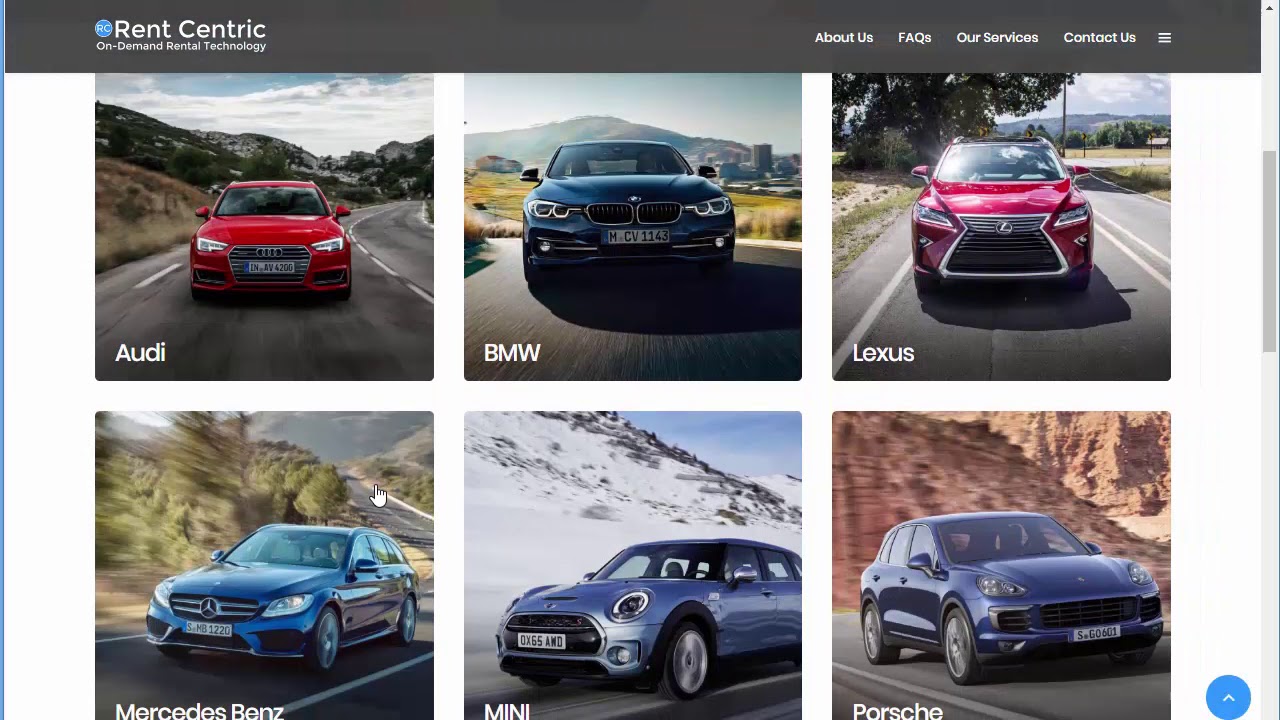This screenshot showcases the Rent Electric car rental company's website, featuring their branding and on-demand rental technology. At the top left of the page, the company name "Rent Electric" is prominently displayed. The navigation bar at the top right, set against a dark blackish-gray background, includes tabs labeled "About Us," "Facts," "Our Services," "Contact Us," and a square icon at the end.

The main content of the page is succinct, highlighting six images of available cars along with their respective brands. The top row features three cars: 
1. An Audi, depicted as a vibrant red car.
2. A BMW, shown in a striking blue color.
3. A Lexus, presented as a red van-like vehicle.

The bottom row also showcases three cars:
1. A Mercedes-Benz, illustrated in a sleek blue color.
2. A Mini, portrayed as a dark blue buggy-like car, uniquely driving amidst snow-covered surroundings.
3. A Porsche, displayed as a dark blue car, standing out as the only vehicle driving in a desert-like setting.

This organized and visually appealing layout provides a clear and engaging snapshot of the car options available through Rent Electric.